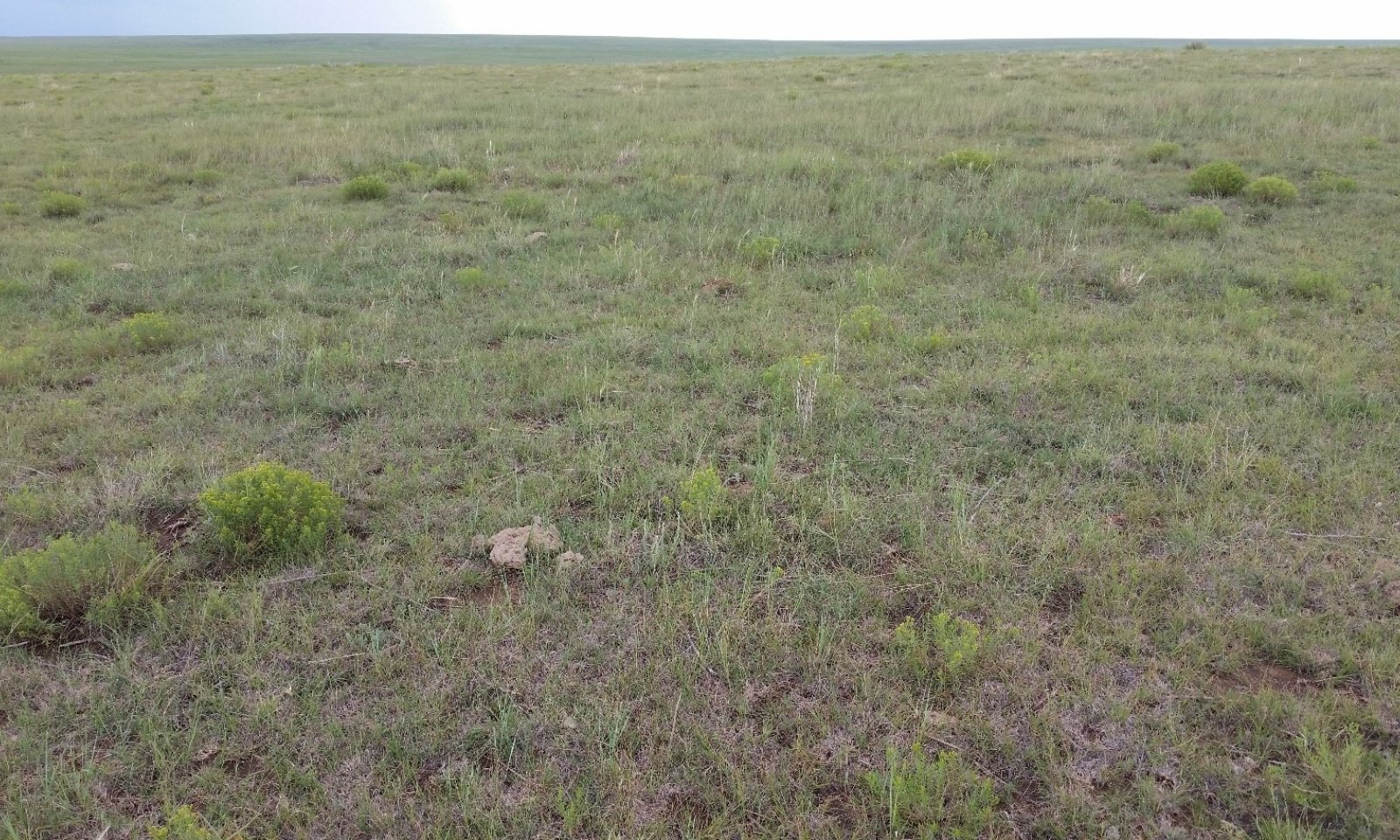The image depicts a vast, flat prairie landscape dominated by sparse vegetation. The grass varies from dry tan to light green, interspersed with a few small bushes and plants that exhibit slightly richer shades of green. The field appears almost endless, with no signs of life such as animals or buildings. Off in the far distance, you can discern a faint line of low hills or a far-off horizon that could be mistaken for the sky. The sky itself is blue but muted, indicating the presence of clouds that diffuse the daylight, leaving the entire scene in a soft, shadowless light. A couple of rocks punctuate the otherwise extensive sea of grass, completing the tranquil and uninhabited atmosphere of this plain landscape.